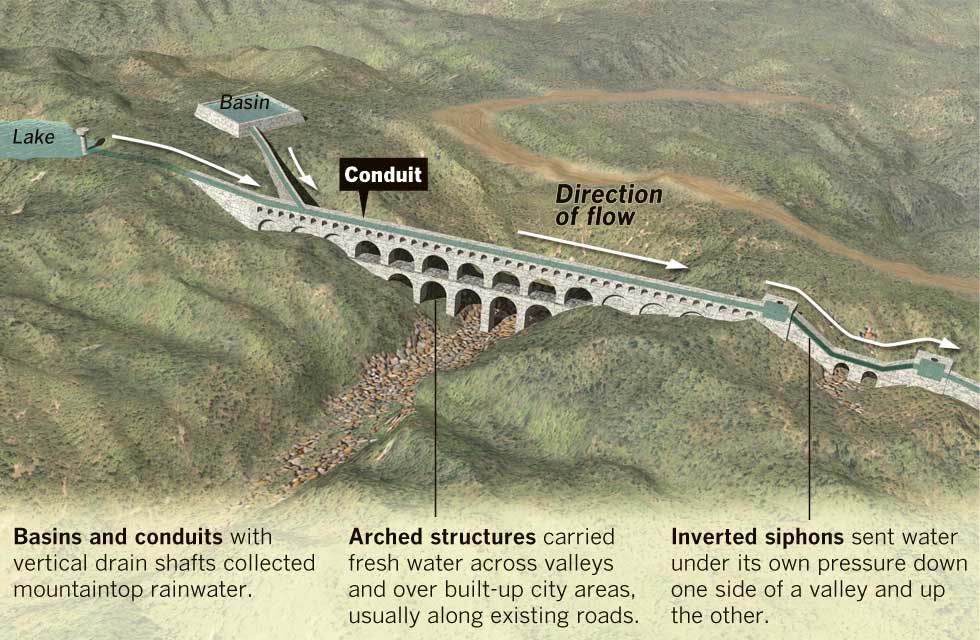This digital poster features a detailed representational drawing at the top, depicting a green terrain with some brown patches. Dominating the scene is a long, light gray bridge spanning an uneven landscape, connecting two masses of grassy land. On one end, the bridge is linked to a lake and a basin. Arrows overlayed on this section indicate a direction of flow pointing to the right, accompanied by text encouraging viewers to "conduct a direction of flow." The bridge is intricate with arched structures suggesting it carries fresh water across valleys and developed city areas, often along existing roads. Additionally, there are inverted siphons designed to transport water under its own pressure down one side of the valley and up the other. The text below this image, organized in three columns against a green background, further explains the functionalities: "Basins and conduits with vertical drain shafts collect mountaintop rainwater," "Arched structures carry fresh water across valleys and over built-up city areas usually along existing roads," and "Inverted siphons send water under its own pressure down one side of a valley and up the other." The entire scene is rendered from a bird's eye view, creating an almost map-like perspective.